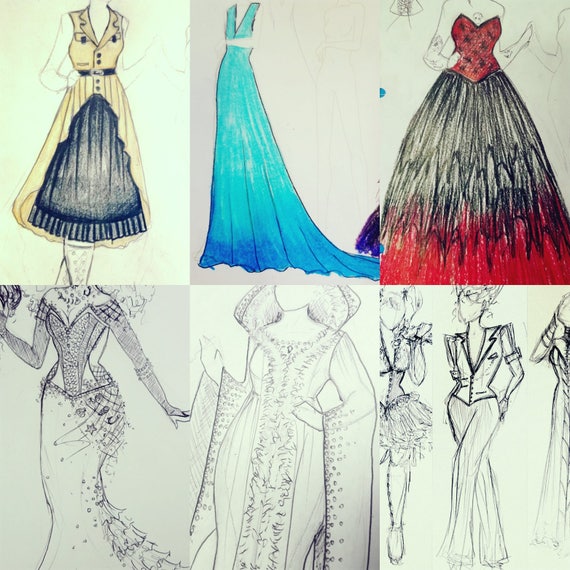The image showcases a set of six intricate sketches of clothing designs, arranged in two rows of three. The top row features colored illustrations, while the bottom row displays monochromatic sketches. 

In the top left corner is a beige v-neck dress that spreads out into a vest-like silhouette. At the center of this dress is a bluish-black splotch forming a triangular pattern. Next to it, in the middle, is a cyan dress embellished with dark blue frills at the hem, creating a gradient, or ombre effect, that darkens towards the bottom. On the top right, there's a striking black and red dress, featuring black stars over a red background on the chest area, with the dress's frills transitioning from black to red at the hem. This dress also incorporates a corset-like bustier design.

Beneath these colored designs are three detailed black and white sketches, presenting intricate patterns and textures for each corresponding design. The leftmost sketch outlines the texture and pattern of a dress without any added color. The center sketch continues this monochromatic trend, detailing the structure of the cyan dress from above. To the right, the third sketch provides a similar black and white outline, depicting what appears to be a pantsuit rather than a dress.

Together, these six images provide a comprehensive look at both the colorful final designs and their detailed conceptual sketches.